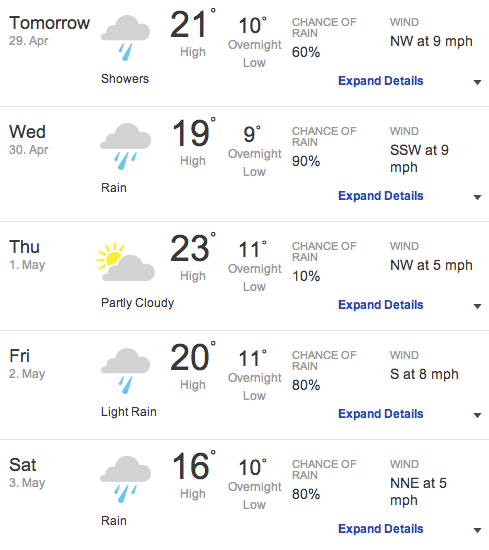Screenshot of a weather forecast displaying detailed information for upcoming days:

- **Tuesday, April 29:** 
  - **Condition:** Showers
  - **Graphics:** Cloud with rain
  - **Temperature:** High of 21°C, low of 10°C
  - **Chance of Rain:** 60%
  - **Wind:** Northwest (NW) at 9 mph

- **Wednesday, April 30:**
  - **Condition:** Rain
  - **Graphics:** Cloud with rain
  - **Temperature:** High of 19°C, low of 9°C
  - **Chance of Rain:** 90%
  - **Wind:** South-Southwest (SSW) at 9 mph

- **Thursday, May 1:**
  - **Condition:** Partly Cloudy
  - **Graphics:** Sun and cloud
  - **Temperature:** High of 23°C, low of 11°C
  - **Chance of Rain:** 10%
  - **Wind:** Northwest (NW) at 5 mph

- **Friday, May 2:**
  - **Condition:** Light Rain
  - **Graphics:** Cloud with rain
  - **Temperature:** High of 20°C, low of 11°C
  - **Chance of Rain:** 80%
  - **Wind:** South (S) at 8 mph

- **Saturday:** (Information not fully provided)

The forecast includes temperature highs and lows, expected weather conditions with corresponding graphics, chance of precipitation, and wind speed/direction for each day.